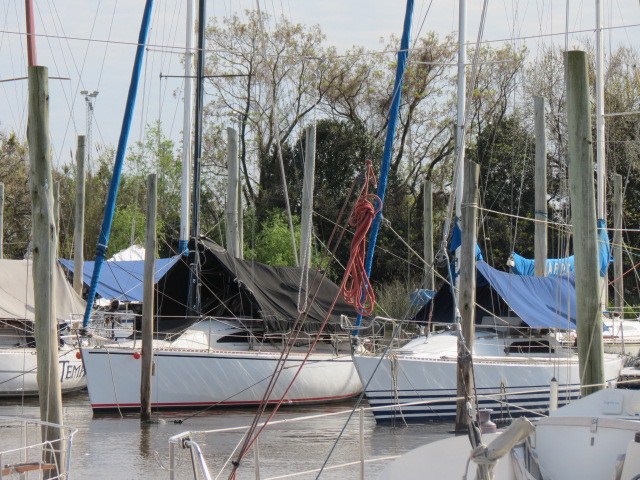This image captures a bustling marina filled with numerous sailboats moored in their slips. The scene is viewed from the perspective of someone standing on a dock or perhaps aboard another boat, looking towards the shore. Dominating the foreground are the white hulled sailboats, accented with varying colors such as red and blue stripes. Their sails are furled, leaving the tall wooden masts and intricate rigging to create a dense, almost chaotic network of lines reaching skyward. Some boats feature protective coverings in an array of colors—black, blue, light blue, and grayish brown—while others are trimmed with black or red. The water in the marina appears dark and grayish, contrasting with the vibrant hulls of the boats. Flanking the marina, the shore is lined with a mix of lush and sparsely leafed trees, suggesting a setting in early spring or late fall. Overarching the entire scene is a pale bluish-gray sky, completing the tranquil yet active atmosphere of this nautical haven.